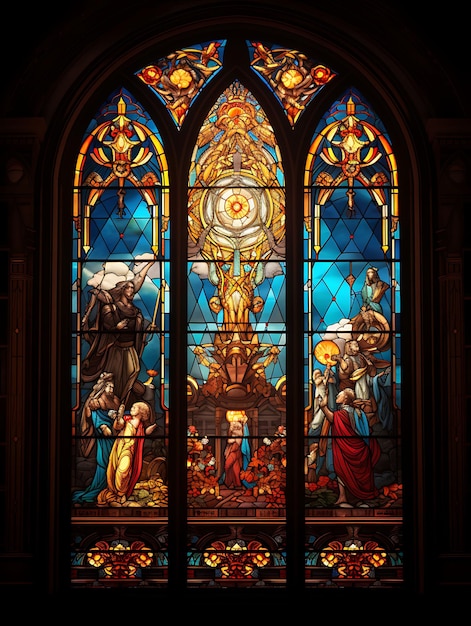The image depicts a striking stained glass window inside a church, composed of three vertical, bullet-shaped columns. The stained glass, framed in a dark midnight blue or black color, is illuminated from within, casting a luminous glow in the otherwise dark surroundings. Each column features intricate biblical scenes with figures dressed in ancient robes of red, brown, and gold. The background predominantly showcases shades of electric blue. The central section is dominated by an elaborate altar adorned with a prominent chalice, occupying the upper two-thirds of the window. Above each column, small interlocking panes add further detail. Throughout the design, one can observe angels, saints, and possibly an angel of death, standing against the vivid tones of blue sky. The carefully curated details and vibrant colors of red, yellow, and white contribute to the piece's religious and ornate aesthetic, culminating in an awe-inspiring depiction of faith and reverence.